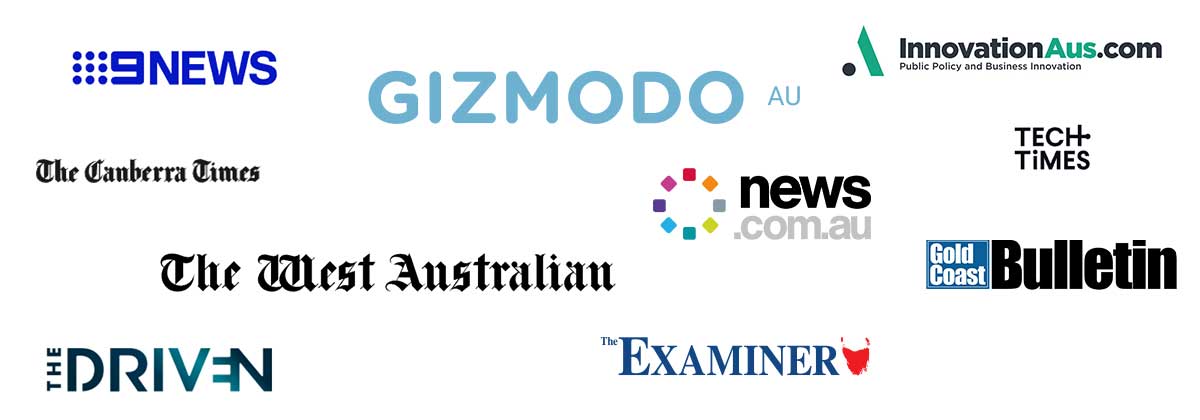This image, set against a white background, features an array of company logos neatly arranged. In the upper left corner, the "Nine News" logo is prominently displayed in navy blue font, accompanied by a grid of nine blue dots arranged in a three-by-three pattern. Directly beneath this, "The Canberra Times" is inscribed in elegant black calligraphy-style text. Following this, "The West Australian" is also presented in a similar calligraphic black font. 

In the bottom left, the logo for "The Driven" is creatively designed, with "THE" positioned vertically, and "Driven" extending horizontally to the right in a gradient of blue to bluish-green and black. Adjacent to this, "The Examiner" is displayed in a navy blue font.

Above "The Examiner," the "News.com.au" logo features a dynamic design of squares forming a rainbow-colored circle. Directly above this, "Gizmodo" is presented in a soft baby blue font. To the right of these elements, the "InnovationAUS.com" logo stands out with "AUS" in green and the rest in black, including the tagline "Public Policy and Business Innovation."

Continuing to the far right, the "Tech Times" logo is arranged with "Tech" placed above "Times," and finally, the "Gold Coast Bulletin" logo completes the array, with "Gold Coast" written in a white font housed within a blue box, next to "Bulletin" in black text.